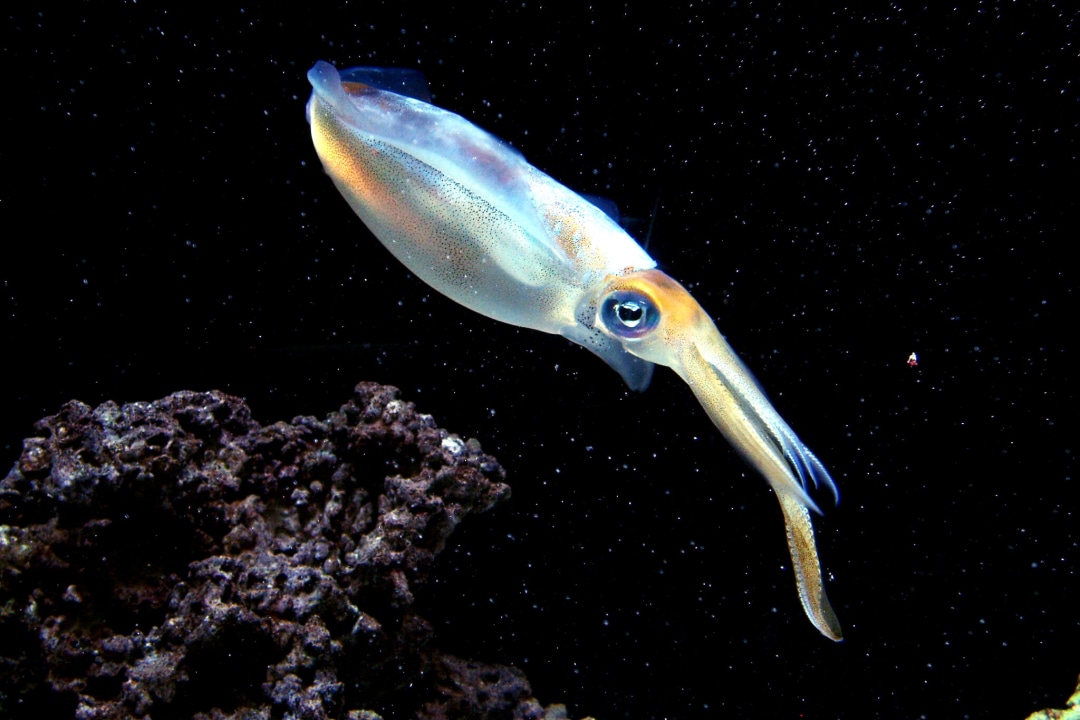In this detailed underwater scene, set against a black background dotted with white specks that resemble stars but are likely air bubbles, we see a vibrant, translucent octopus in a side profile positioned centrally. The octopus boasts a striking blend of colors: clear blue with accents of orange and yellow, a blue eye, glowing yellow underneath, and translucent white tentacles with blue tips. In the bottom left corner, a dark coral – almost rust or bronze in color – adds texture to the scene. The overall setting, characterized by its profound darkness, suggests it was captured in the deep sea. The diverse color palette includes shades of black, white, brown, purple, yellow, orange, red, and blue, enhancing the intricate details of the octopus and the surrounding environment.